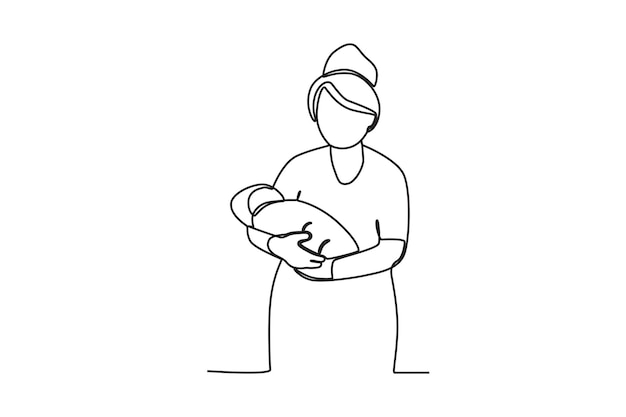This black-and-white line drawing depicts a featureless woman, possibly a nurse or mother figure, cradling a swaddled infant in her arms. The woman is dressed in a short-sleeved gown and wears gloves. Her head is adorned with what appears to be a nurse's cap or a hairstyle with a band resembling a bun. The baby, nestled in the crook of her right arm, has a cap on its head and is wrapped securely in a blanket. Both the woman and the infant have blank, round faces with no discernible facial features. The simplistic and somewhat crude sketch seems to blend the woman's dress into the white or transparent background, giving it an ethereal quality. The drawing style is reminiscent of a single, uninterrupted stroke, further emphasizing its minimalistic nature.